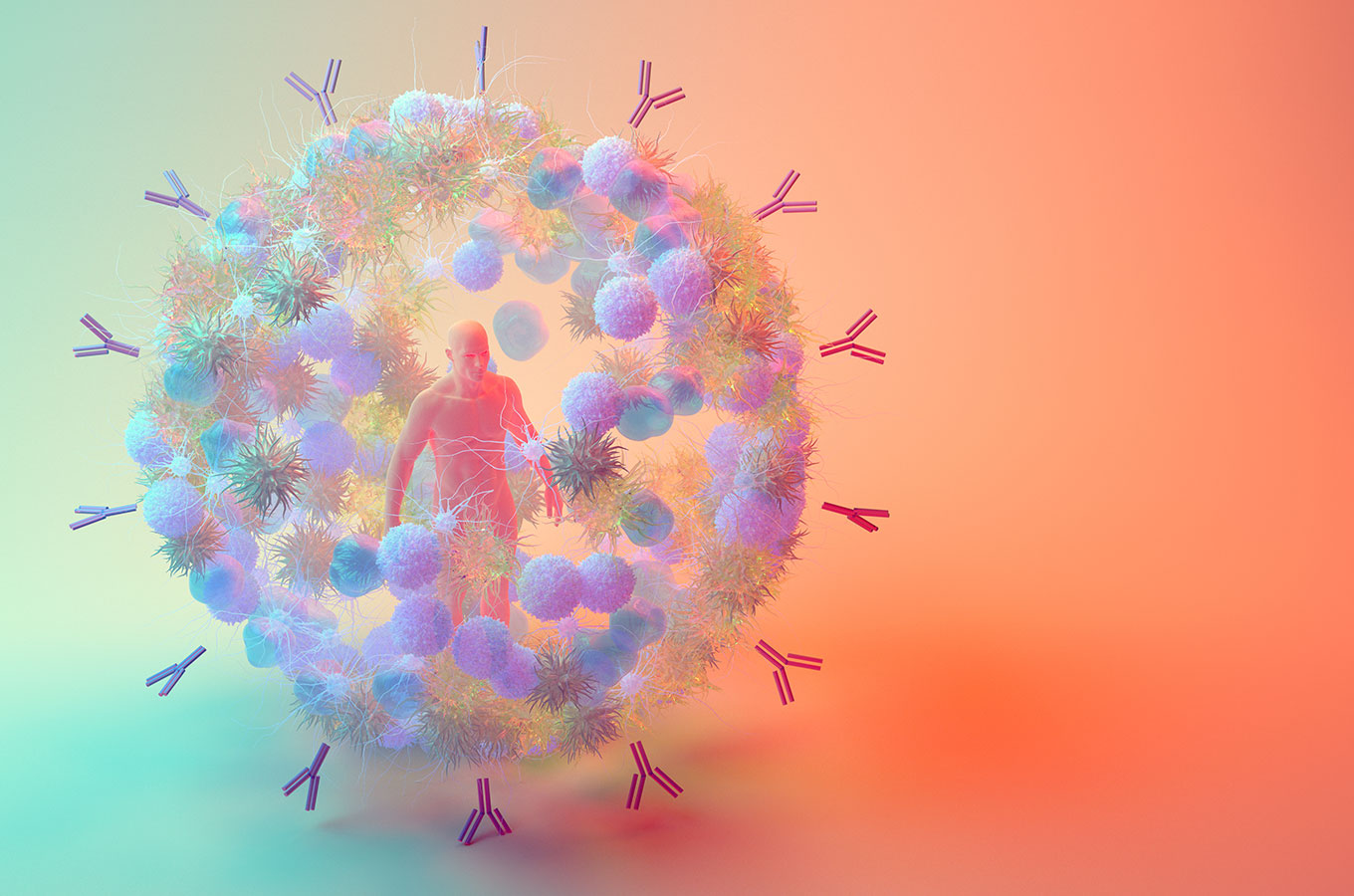The image is a horizontal rectangular abstract scientific illustration with a vibrant gradient background. About two-thirds of the right side features a rich orange hue, while the left side transitions into an aqua or very light greenish-blue color. Central to the image is a circular structure composed of numerous smaller circular elements, displaying a spectrum of colors including purples, dark aqua, and touches of orange. Encircling this structure are Y-shaped formations that appear to be part of a scientific visualization.

Within the central circular design, there seems to be a 3D representation of a human figure, depicted as nude and bald, standing amidst a swarm of spherical and cloud-like shapes that may represent molecules or particles. These particles vary in shades of pink, orange, and dark pink, harmonizing with the background tones. The entire scene appears to represent some form of biological or disease-related interaction, making it suitable for a scientific poster illustrating the effects of a disease on the body.